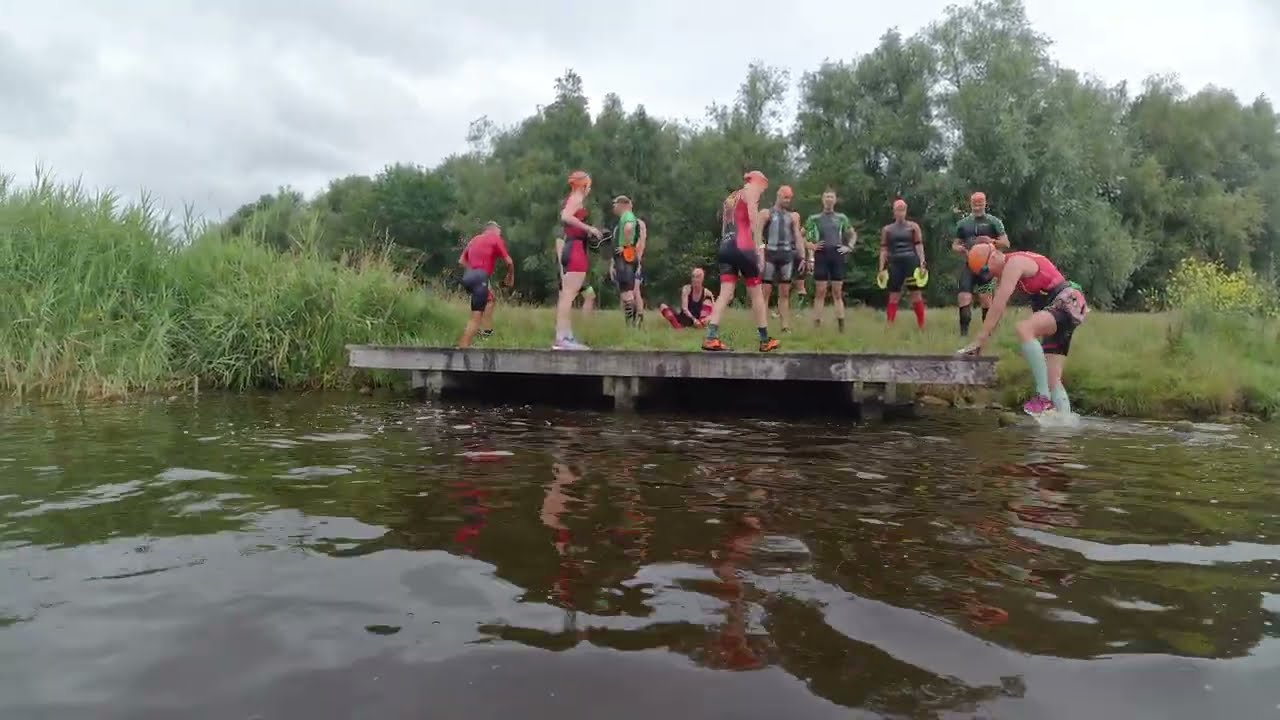The color photograph, captured in landscape orientation, provides a vivid scene of a group of people gathered around a murky brownish pond. Central to the image is a wooden dock or platform, on which three individuals are standing. A young boy, clad in a helmet and wetsuit, is seen climbing out of the water onto the dock. The people on the dock are dressed in either tank tops and shorts or full wetsuits, suggesting they have been engaging in water activities.

On the grassy bank surrounding the pond, which is populated with tall reeds and weeds, six men and a child can be observed. These individuals are mostly in red tops and black shorts, possibly indicating team attire, hinting at a competitive event. They are either standing, facing different directions, or sitting down, with some players holding circular objects, likely part of their game gear.

The backdrop features a lush green field transitioning into a dense line of trees under a cloudy gray sky, enhancing the naturalistic and serene setting of the scene. Taken from what could be a drone or an eye-level perspective from the pond, this photograph captures a detailed, representational view of a lively yet tranquil outdoor gathering.